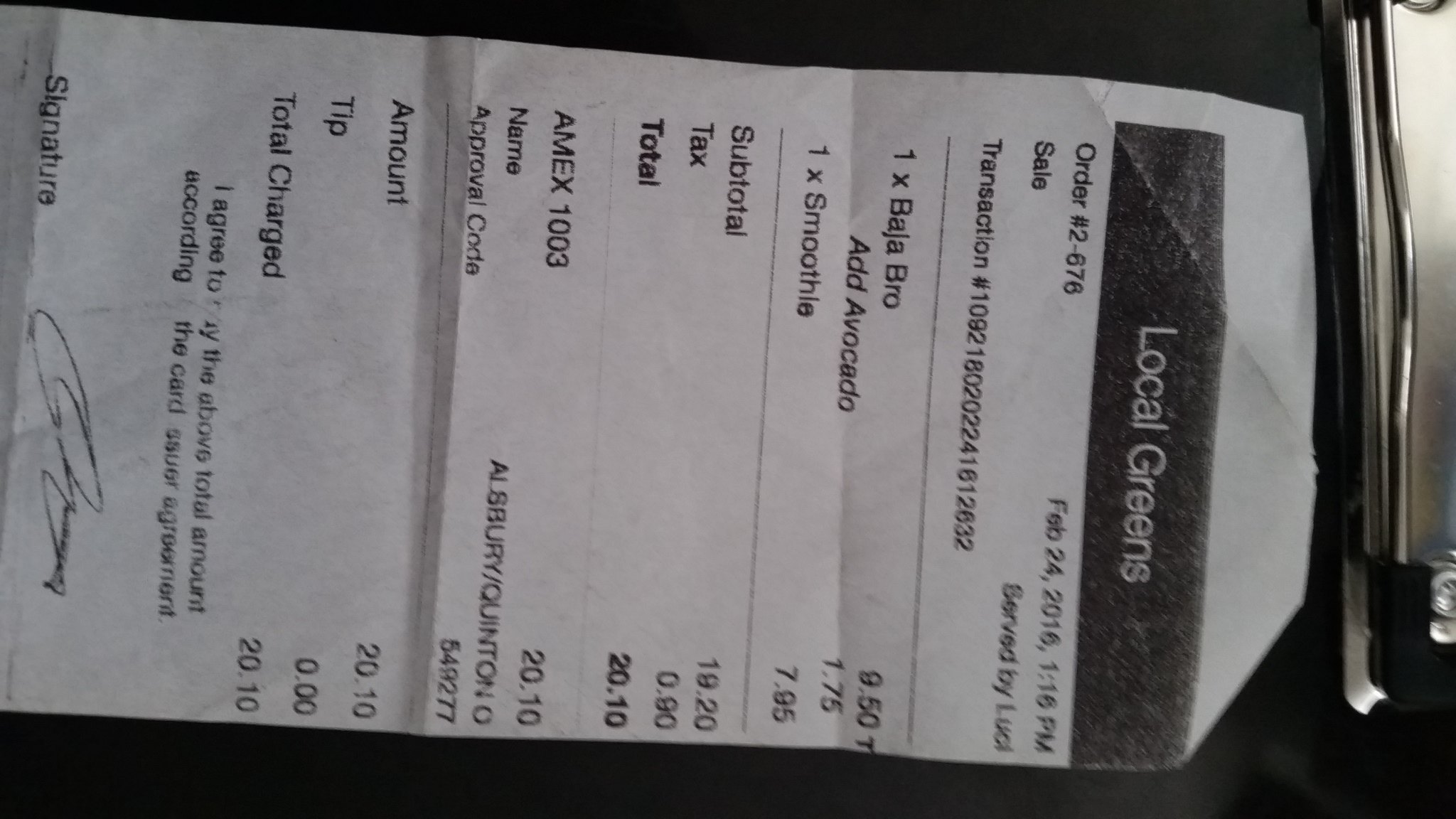The black and white photograph showcases a receipt or sale slip, lying horizontally in the frame. To correctly view and read the document, it should be rotated 90 degrees counterclockwise. On what is currently the right side of the image, there's a metallic edge resembling a clipboard or hole punch, indicating that the receipt might have been attached to something. 

The receipt is from a place named "Local Greens" with order number 2-676, dated February 24th, 2016 at 1:16 p.m. It records a transaction executed by an employee named Lucy (spelled L-U-C-I). The order comprises one "Baja Bro" priced at $9.50, an added avocado for $1.75, and one smoothie costing $7.95. The subtotal before tax is $19.20, with an additional $0.90 tax, bringing the total to $20.10.

Payment was made using an American Express card ending in 1003. The name associated with the card is Alsbury/Quinton O. An approval code is also mentioned, alongside the total amount charged. No tip was added, finalizing the total charge at $20.10. The receipt also includes a standard agreement statement concerning the total amount and cardholder's agreement, followed by a signature line and the cardholder's signature.